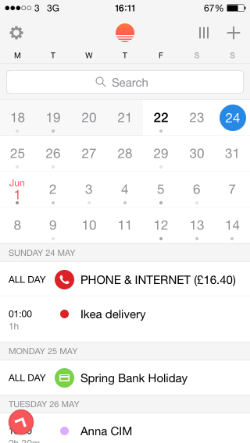Here's a cleaned up and detailed caption for the screenshot image:

---

The screenshot displays a smartphone screen, starting with the status bar at the top. The bar includes three black dots followed by two gray ones, indicating signal strength. It also shows "3G" connectivity, the time "16:11," and a battery level of 67%.

Below the status bar, there is a gray cogwheel representing settings, and an orange and pink circle icon. Adjacent to it are three horizontal gray lines (menu icon) and a gray plus sign. Next, the days of the week from Monday to Sunday are listed.

Further down, there is a white search box with a gray magnifying glass icon and the word "search" inside. Below that is a calendar view featuring dates. The dates 18th to 21st of the current month are shaded in gray, with the 22nd highlighted in black. The 23rd is grayed out, while the 24th is circled in blue with white digits. Dates from the 25th to the 31st are also in gray. June 1st is marked in red, and dates up to June 14th are gray.

On the calendar, it says "Sunday 24th May" followed by "all day, phone and internet, £16.40" in black text. A red circle with a white phone icon is placed between "all day" and "phone and internet." Below that is a notation for "one hour" marked by a red dot, and “Ikea delivery” in black text. Next, it mentions "Monday 25th of May," designated as an "all day spring bake holiday" with a green card icon beside it.

Further down still, it says "Tuesday 26th of May" with a red circle containing a white arrow, and a purple circle denoting "Anna C.I.M." This section of the screenshot is clear and easy to read with all elements clearly labeled.

---

This caption provides a detailed and structured description of the elements visible in the screenshot.